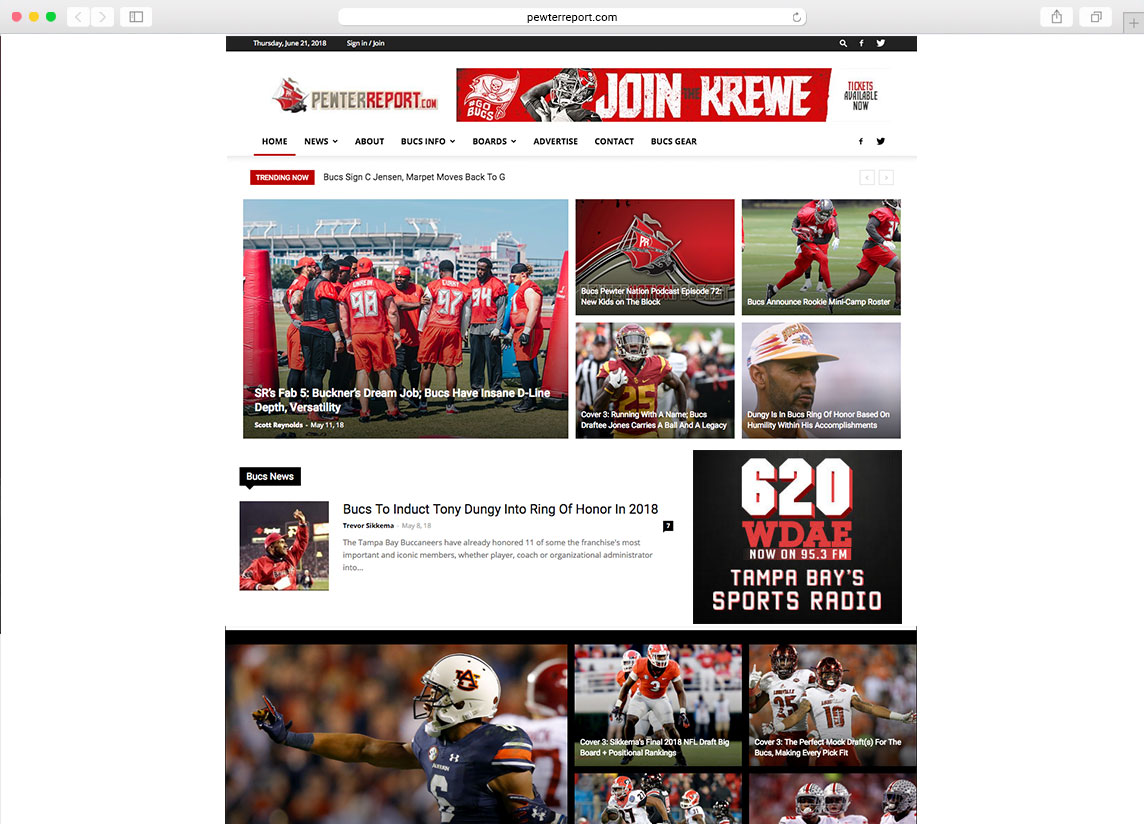This detailed screenshot captures the vibrant interface of PewterReport.com, a website dedicated to football, with a dominant focus on the Tampa Bay Buccaneers. The screenshot, taken on a Mac browser, displays the website's header prominently, featuring the title "Pewter Report" and a stylish pirate ship logo adorned with red sails and flags on the left side.

At the top of the page, there is a catchy banner reading "Join the Krewe," stylized with a 'K' instead of a 'C,' accompanied by a Tampa Bay Buccaneers pirate flag and an image of someone saluting tickets. A comprehensive menu bar lies beneath the header, offering navigation options including Home, News, About, Bucs Info, Boards, Advertise, Contact, and Bucs Gear, emphasizing the site's primary focus on the Tampa Bay Buccaneers.

Below the main banner, a section titled "Training Now" features an image from a Buccaneers training camp. This scene includes players engaging with heavy bags, set against the stadium backdrop. The players are depicted in their jerseys and shorts, sans pads, indicating a training or practice session.

To the right of this training camp image is a four-photo overlay grid. While the text is unreadable, visual elements include the Buccaneers logo and images of:
- A player catching a ball.
- Another player, seemingly a USC athlete, suggesting a draft pick.
- A coach wearing a hat.

Further below, the page highlights a significant photograph of Tony Dungy being inducted into the Buccaneers' Ring of Honor in 2018, celebrated during a special moment.

Adjacent to this, an advertisement for 620 WDAE, a known Tampa Bay Sports Radio Station, is prominently displayed, establishing a local sports media connection.

The lower section of the page features a similar photo grid format, displaying various college football images, arranged in one large photo with four smaller ones to the right. These images capture different collegiate teams, yet maintaining the overall football-centric theme of the site.

In summary, this screenshot intricately showcases PewterReport.com's dedication to football, particularly emphasizing the Tampa Bay Buccaneers, with a visually engaging and content-rich layout focused on delivering a comprehensive football experience.